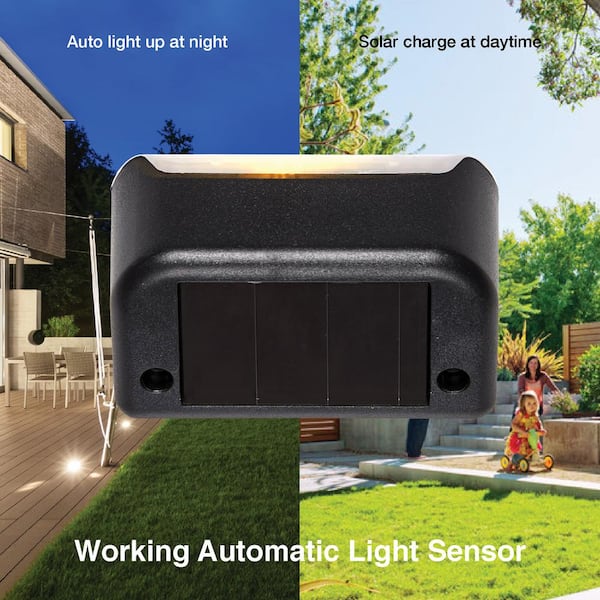The image is an advertisement for a light sensor, presented in a square format with two vertical background photographs side by side. The left half of the image depicts a nighttime backyard scene, featuring a dark blue sky, a building with a deck, and some green grass. White text at the top-left reads "Auto light up at night."

The right half of the image showcases a daytime backyard scene. It depicts bright sunlight, a green yard, trees, a little girl riding a bike, and her mother sitting on some concrete steps. Overlayed text in black at the top-right reads "Solar charge at daytime."

In the center of the image, superimposed over both background photographs, is a large, rectangular, black object with rounded corners and a drop-down panel, resembling a light sensor with a solar panel on top. Across the bottom middle of the image, spanning both the night and day scenes, is white text that reads "Working automatic light sensor."

The overall style combines photographic realism with graphic design elements and text to highlight the dual functionality of the light sensor in various lighting conditions.